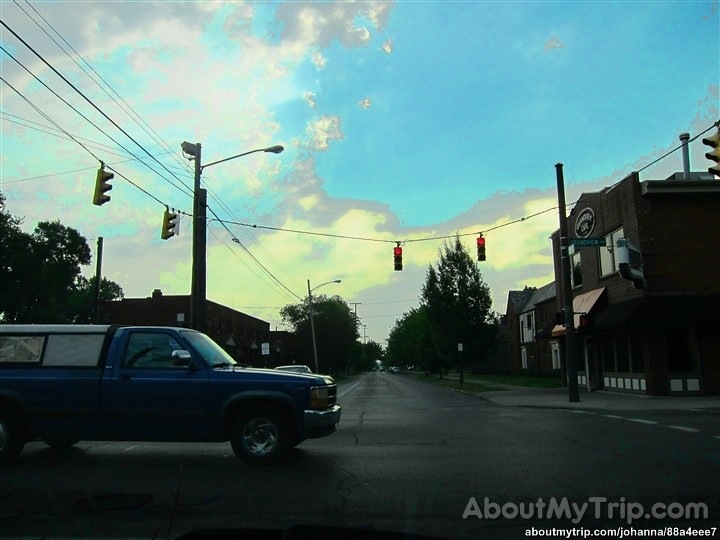The photograph captures a quaint intersection in a small town, viewed from the perspective of someone sitting in a car at a red light. The scene is dominated by a blue pickup truck with a white camper shell, crossing the road from the left side. The early morning sky is light blue with wispy clouds and the sun lies low on the horizon, casting a gentle morning hue. The quiet streets are lined with brick buildings, sidewalks, and scattered trees, giving off a charming, almost desolate small-town atmosphere. Two red stoplights can be seen hanging above the intersection, reinforcing the stillness of the moment. The image has a slightly off-color, monochrome overlay, adding a vintage feel to the scene. In the bottom right corner, the website aboutmytrip.com along with "aboutmytrip/Johanna/some ID number" is clearly visible, marking this image as part of a travel documentation series.